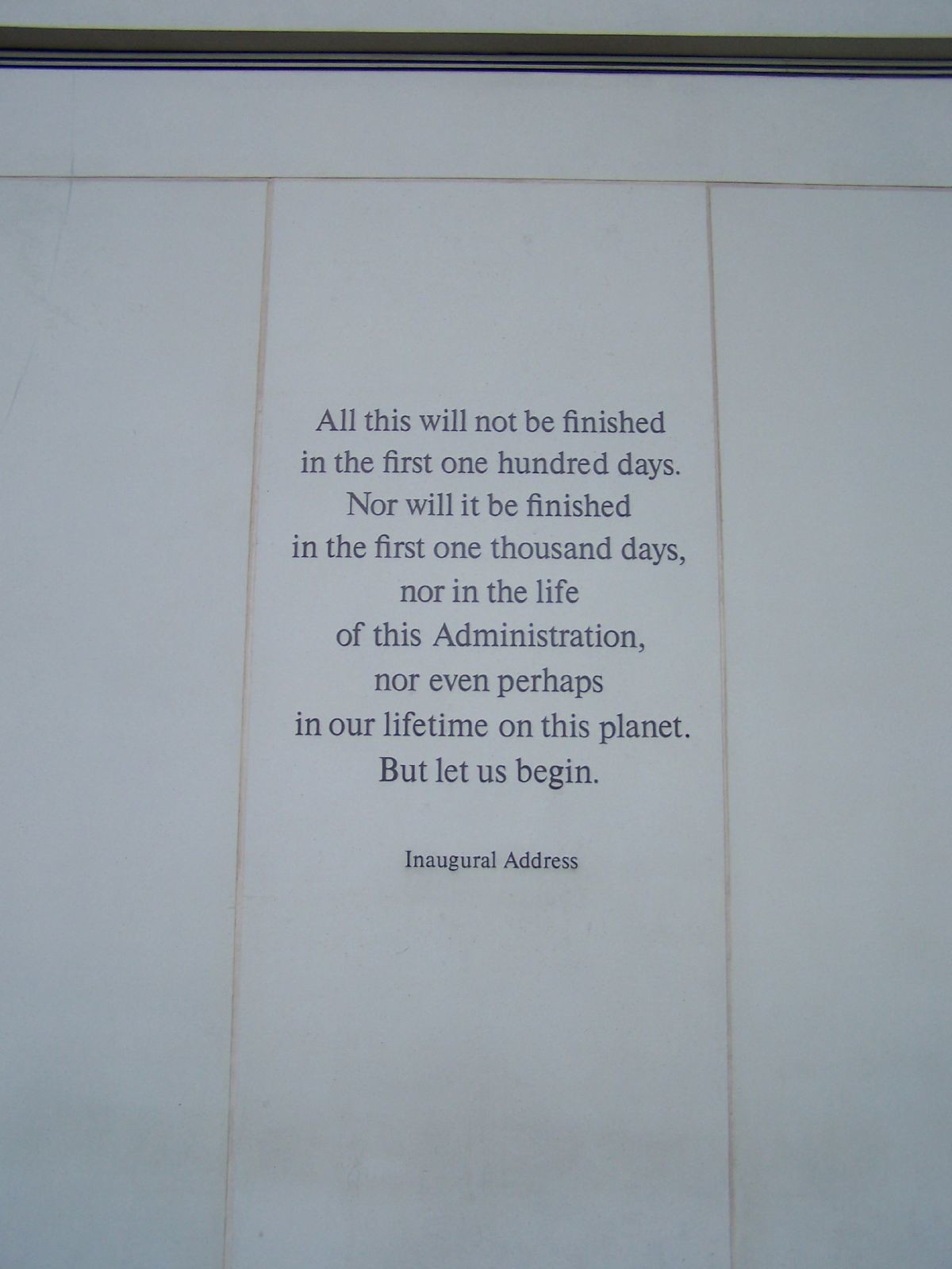The image depicts a singular object centered within the frame: an engraved text on a grayish barrier, which could either be concrete or marble. The text appears against a white to whitish-gray background that is bordered by an orangish or brown trim at the top, adding a subtle touch of black trim horizontally. The inscription reads, "All this will not be finished in the first 100 days, nor will it be finished in the first 1,000 days, nor in the life of this administration, nor even perhaps in our lifetime on this planet, but let us begin." It is noted as an "Inaugural address," seemingly related to a presidential speech. The overall aesthetic is simple yet has a historical or governmental vibe, with the text being the focal point of the image. The architecture hints at an older style, though no specific time period or location can be determined.